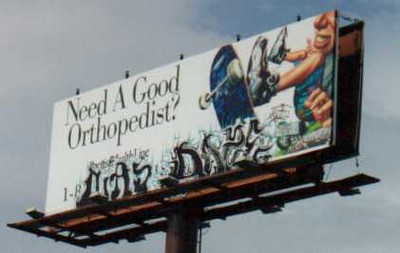This photograph captures a high-mounted billboard, supported by a sturdy, brown-colored cylindrical metal post. Encircling the billboard on both sides is a metal U-shaped walkway, designed for access and maintenance. The billboard itself features a white background and an image of a person falling off a blue skateboard with white wheels. The figure, donning white sneakers, is depicted mid-fall, leaning backwards. The text on the billboard reads, "Need a good orthopedist?" However, the area typically reserved for a contact number has been defaced with gray and black graffiti that spells "LASDAZE." The scene is set against a backdrop of a clear blue sky with a scattering of light clouds.